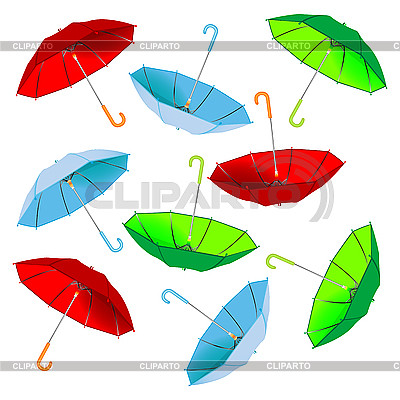This graphic image, appearing to be a piece of clipart, is marked by the watermark "Clipart O" horizontally across its center in faint, transparent grey. The watermark is also repeated in thin, approximately half-centimeter thick banners at the top and bottom of the image. The main illustration features nine umbrellas in various positions, including upright, diagonal, and upside down, as if they are falling randomly from the sky. The umbrellas are evenly distributed among three colors: red, blue, and green, with three umbrellas in each color group. Each umbrella has a silver stem and a handle that matches the color of its canopy.